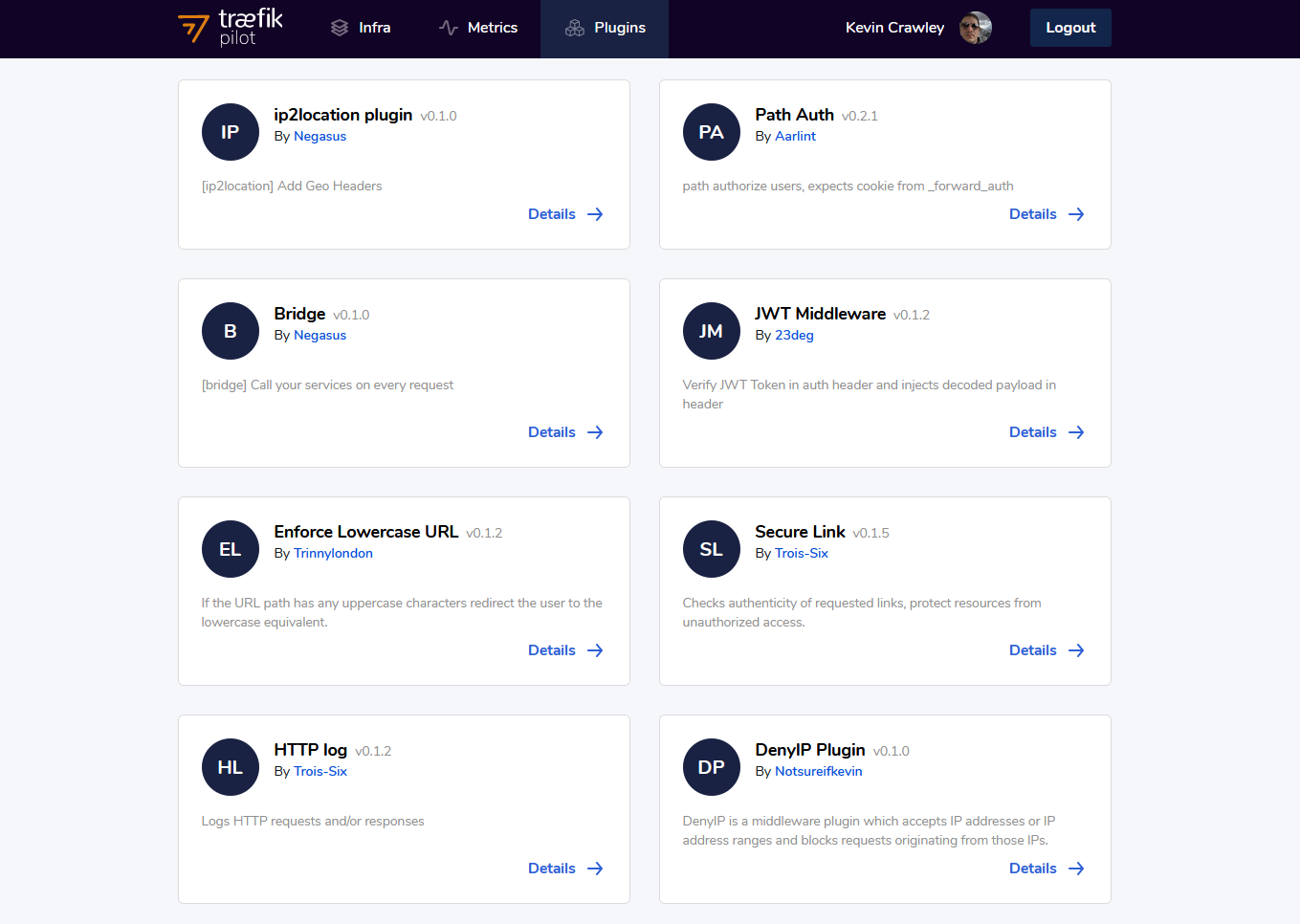The image displays a webpage layout with the header section containing several tabs: "Infra," "Metrics," "Plugins," and "User Profile," with the profile named Kevin Crowley, along with a blue "Logout" button. 

On the top left, there's a tab labeled "Traffic Pilot," featuring an orange logo. The active tab on the page is "Plugins," showcasing a grid of 8 plugins organized in 2 columns and 4 rows.

1. **IP2 Location Plugin**
   - **Version**: 0.1.0
   - **Author**: Negasas (displayed in blue)
   - **Description**: Geo Headers

2. **Bridge**
   - **Version**: 0.1.0
   - **Author**: Negasas
   - **Description**: Call your service on every request.

3. **Enforce Lowercase URL**
   - **Version**: 0.1.2
   - **Author**: Tiny London
   - **Description**: If your URL path has an uppercase character, redirect the user to the lowercase equivalent.

4. **HTTP Log**
   - **Version**: 0.1.2
   - **Author**: Troy6
   - **Description**: Logs HTTP requests and/or responses.

5. **Pet Auth**
   - **Version**: 0.2.1
   - **Author**: Elint
   - **Description**: Authorizes users to expect cookies from forward auth.

6. **JWT Middleware**
   - **Author**: 23Deck
   - **Description**: Verifies JWT token in auth header and injects the decoded payload in the head.

7. **Secure Link**
   - **Version**: 0.15
   - **Author**: Troy6
   - **Description**: Checks the authenticity of the requested link, protecting resources from unauthorized access.

8. **DynIP Plugin**
   - **Author**: Notsureifkevin
   - **Description**: Middleware plugin that accepts IP addresses or IP address ranges and blocks requests originating from those IPs.

The organized presentation showcases detailed information about each plugin, including its version, author, and functionality.